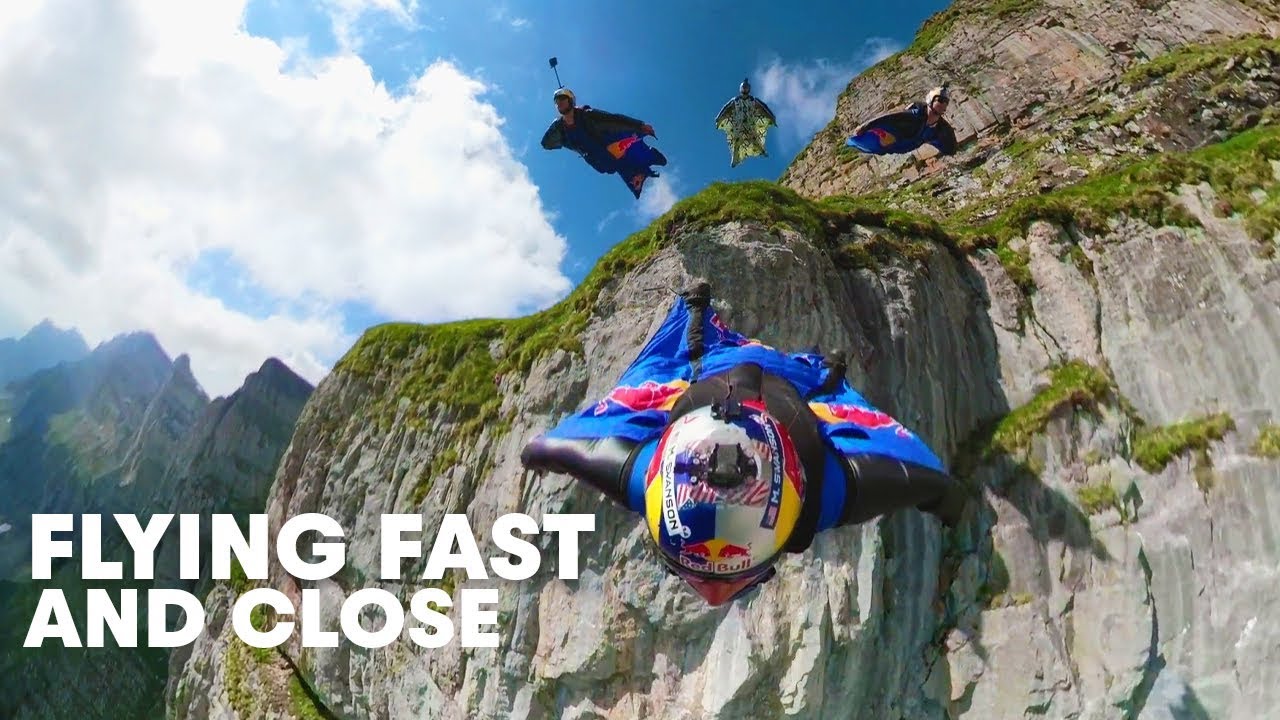The image captures a thrilling skydiving moment with four divers leaping from a mountain cliff. The cliff in the background is a rugged gray structure contrasting vividly with the clear blue sky and a broad, white cloud. The divers, all wearing wingsuits that resemble flying squirrels' webbed limbs, appear to be captured in mid-air. Three of the skydivers are wearing blue and black suits, while the fourth diver, positioned farthest from the camera, sports a green or beige suit. The closest diver to the camera dons a Red Bull-sponsored helmet with a visible GoPro, and their name, "M. Swanson," is written on the helmet. The image features the text "FLYING FAST AND CLOSE" in bold, white, capital letters at the bottom left, underscoring the intensity and proximity of the jump.